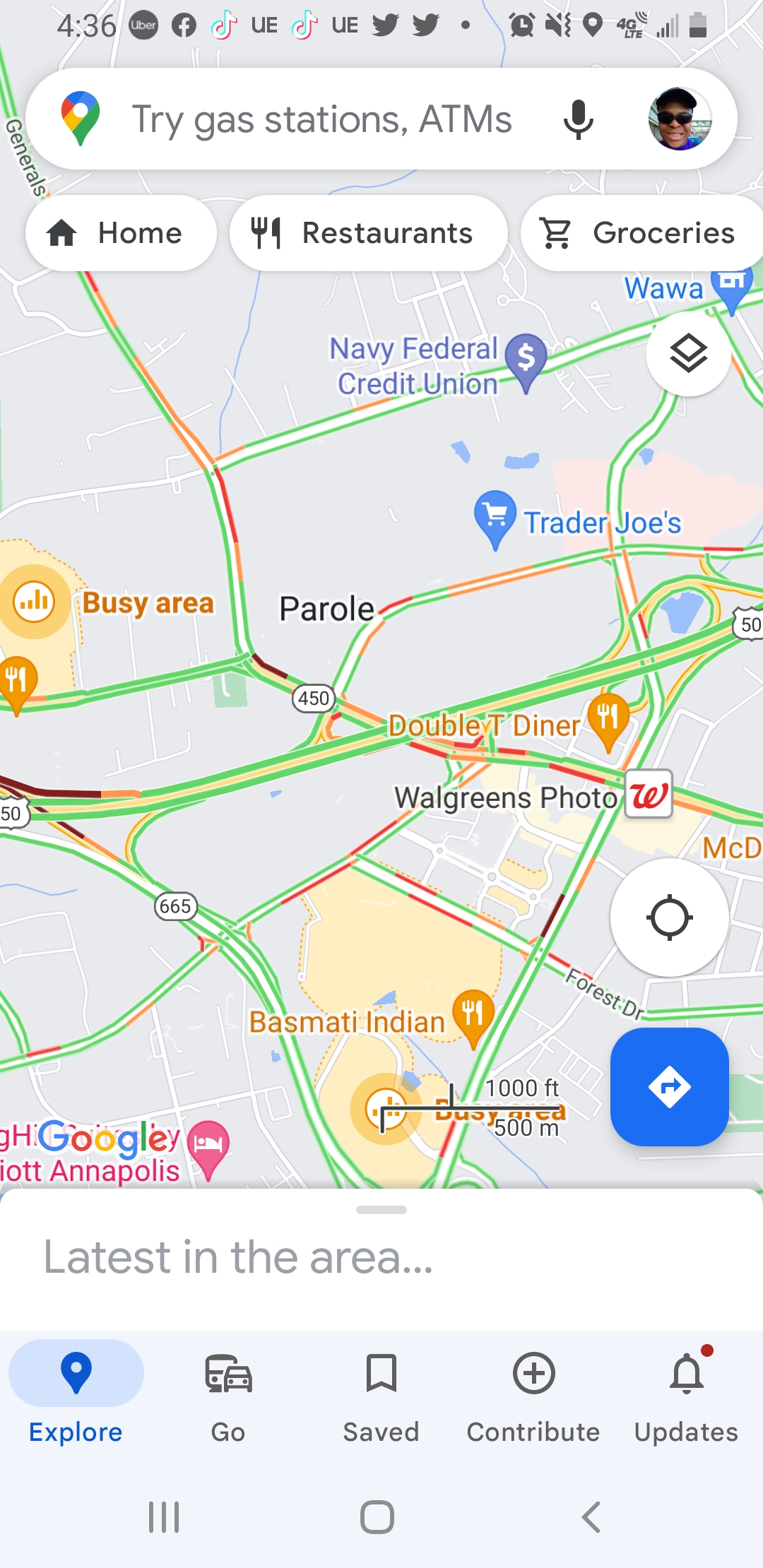The photograph captures a detailed screenshot from a Google Maps application on an Android cell phone. The top left corner of the screen displays a time of 4:36, and various notification icons are visible, including those for Facebook, TikTok, Uber, Uber Eats, Twitter, and an alarm clock. The search bar contains the text "TriGas Stations ATM" with an option to speak into the microphone and an avatar icon next to it. Below the search bar, quick-access icons are labeled Home with a house icon, Restaurants with a fork and knife icon, and Groceries with a shopping cart icon. 

The background map depicts a busy area with multiple labeled locations including Trader Joe's, Walgreens Photo, Parole, Moss, Motty Indian, Wawa, Navy Federal Credit Union, Double Diner, McDonald's, and Basamonte Indian. Notably, the map shows the Marriott Annapolis indicating that the area could potentially be Annapolis, Maryland. Green and red routes are outlined, indicating traffic conditions. 

At the bottom of the screen, tabs for Explore, Go, Save, Contribute, and Updates are present, along with a home button and a back icon, confirming it is an Android device. This screen does not indicate an active destination search but rather shows the general overview or home screen of the Google Maps application.